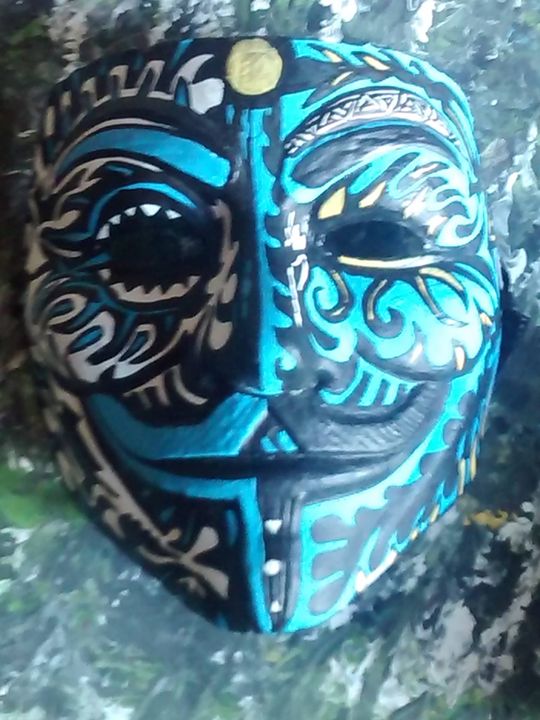This image features an up-close view of a vividly hand-painted mask set against an abstract, smeared background of white, green, and black with hints of gray. The mask dominates the center of the frame, drawing attention with its striking tribal motif and primarily blue hues. The mask’s left side is painted in a darker, oceanic blue, accentuated with looping white swirls outlined in black around the eye. The right side features a lighter sky blue coloration, with white and blue projections encircling the eye cutout, adding a jagged detail to the design.

A gold circle, about the size of a dime, is prominently placed at the center of the mask. The area around the eyes includes a mix of black and white tribal designs, particularly noticeable on the upper right eyebrow which has alternating black and white triangles. The lips of the mask feature a dichotomy: a section painted in a bluish hue on the left and outlined in black on the right, contributing to the overall intricate aesthetic of the mask. This detailed decoration is the main focus of the photograph, creating a captivating visual against the harmonious yet chaotic backdrop.